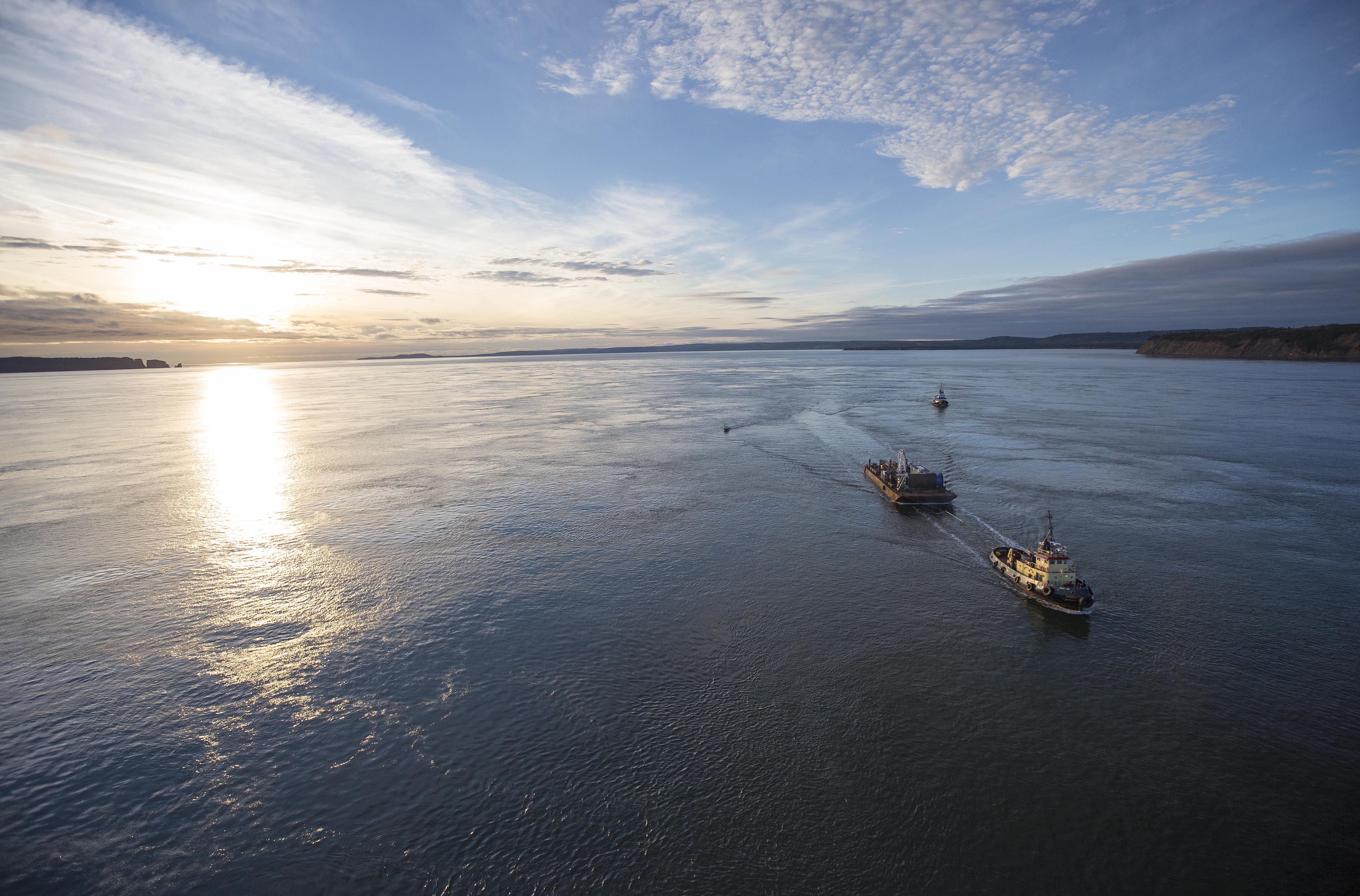This overhead photograph captures the serene beauty of a sunset or sunrise over a tranquil lake. The sun, positioned on the left-hand side of the image, bathes the scene in warm, golden light. The sky above is a radiant blue adorned with white, puffy clouds and some darker, gray clouds scattered across the horizon. The calm waters of the lake reflect the sky and the sun's glow, adding to the image's tranquil atmosphere. 

Dominating the lower part of the image, two tugboats appear to be pulling a barge. The lead tugboat, with its white superstructure and bulky, square shape, stands out clearly, while the barge it pulls is a copper-brown color, although specific details are hard to discern. Off in the distance, a smaller boat can be seen. Several buoys float in the water, serving as navigational markers. 

The overall scene is devoid of any visible land except for a hint of shoreline that juts out into the water, possibly indicating an inlet. The clear, beautiful water and the seamless blend of sky and water in the background enhance the image's captivating and tranquil essence.